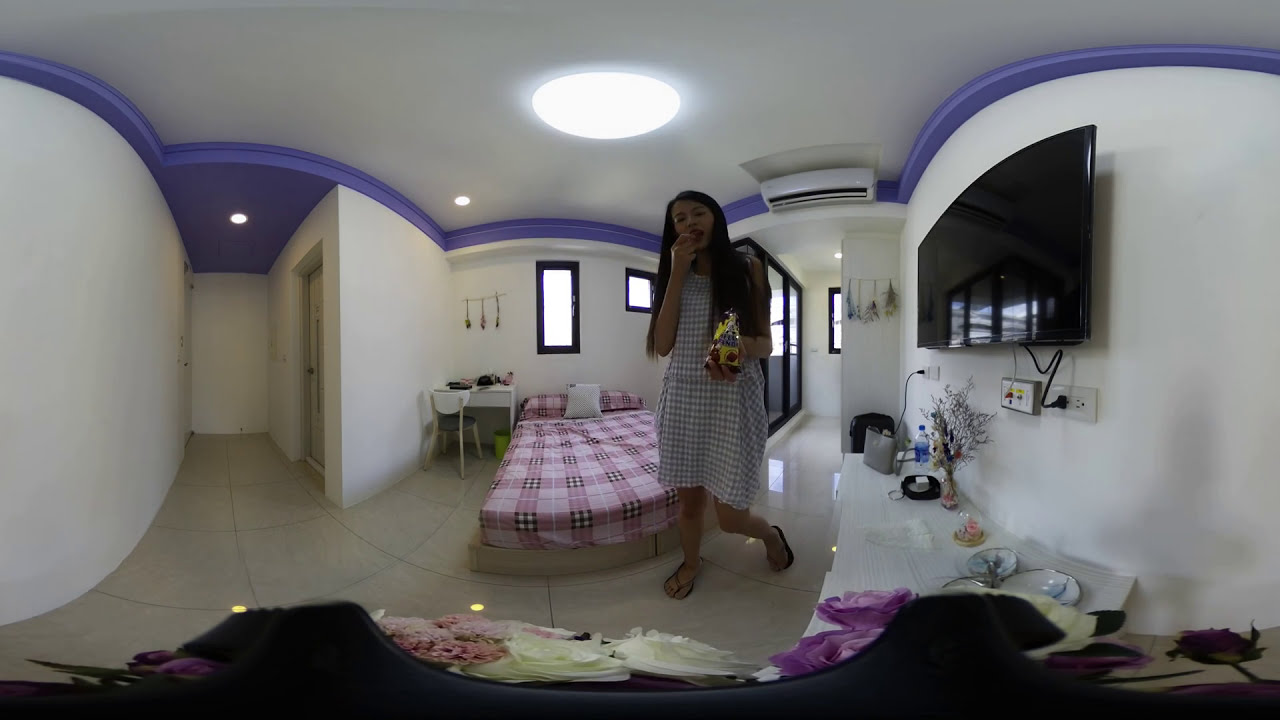The image portrays a young girl with long dark hair, wearing a gray and white checkered dress and flip-flop type sandals, standing in an indoor room with a modern design. The girl, who has Asian facial features, is captured in the center of the photo, holding a yellow bag of chips with text in blue, suggesting she is enjoying a snack. She stands in front of a platform bed that is covered with pink, black, and white plaid bedding, complemented by a white cushion and two pink pillows.

The room's white walls are highlighted with a periwinkle blue trim at the top, and multiple glass windows with black borders allow natural light to filter in. To the right of the girl, a large flat screen TV is mounted on the wall, next to which various electronics are plugged in. A nightstand, a white and gray study table with a blue and white chair, and a green waste paper basket beneath the table contribute to the room's decor. The floor is laid with ceramic tile, enhancing the clean and modern aesthetic.

On the left side of the image, a closed door suggests entry to another room, while shelves holding a vase of colorful flowers, a purse, a water bottle, and several other items are visible. The ceiling features a white vent, various light fixtures, and an AC unit, with the design incorporating blue sections that add a vibrant touch to the overall setting. Wall hangings and other decorations add personality and warmth to the girl's personal space.